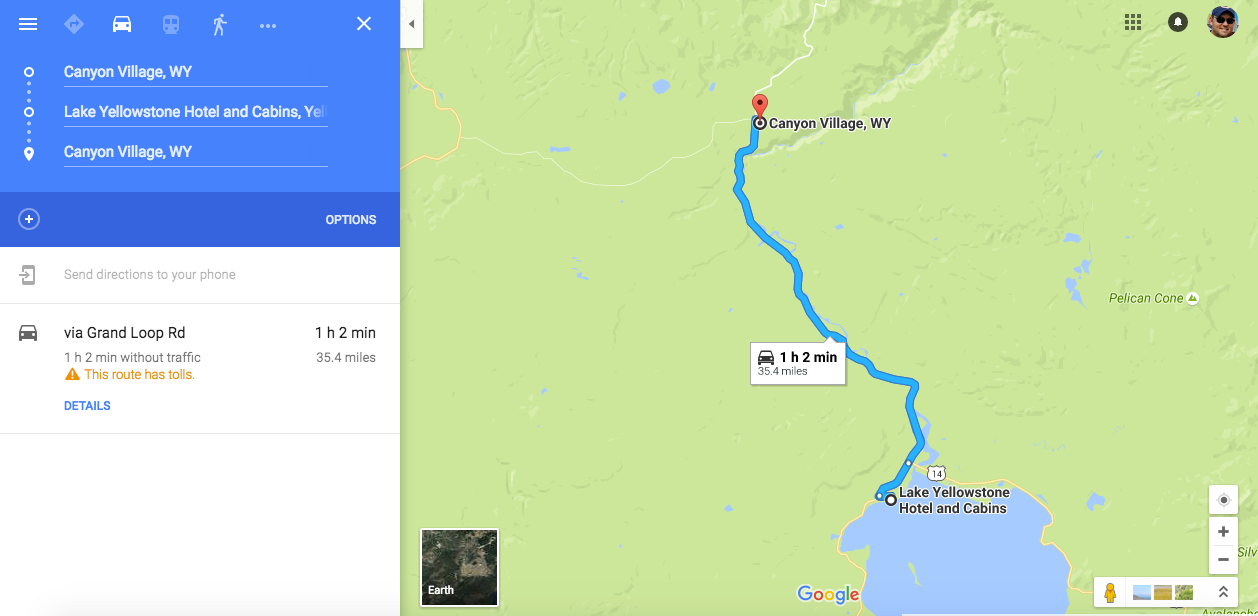The image features a couple of screenshots captured from a smartphone, showcasing a map from Google Maps. On the right side of the image, the detailed map section displays a prominent green landscape interspersed with a noticeable blue patch of water towards the bottom, likely a lake. A planned car route is highlighted on the map, indicating that the journey from Lake Yellowstone Hotel and Cabins to Canyon Village in Wyoming is estimated to take one hour and two minutes. The destination, Canyon Village, is marked with a red pin. On the left side of the image, there is a blue border with white text beneath it, which reiterates the journey details in a different layout, indicating the start at Lake Yellowstone and the endpoint at Canyon Village.